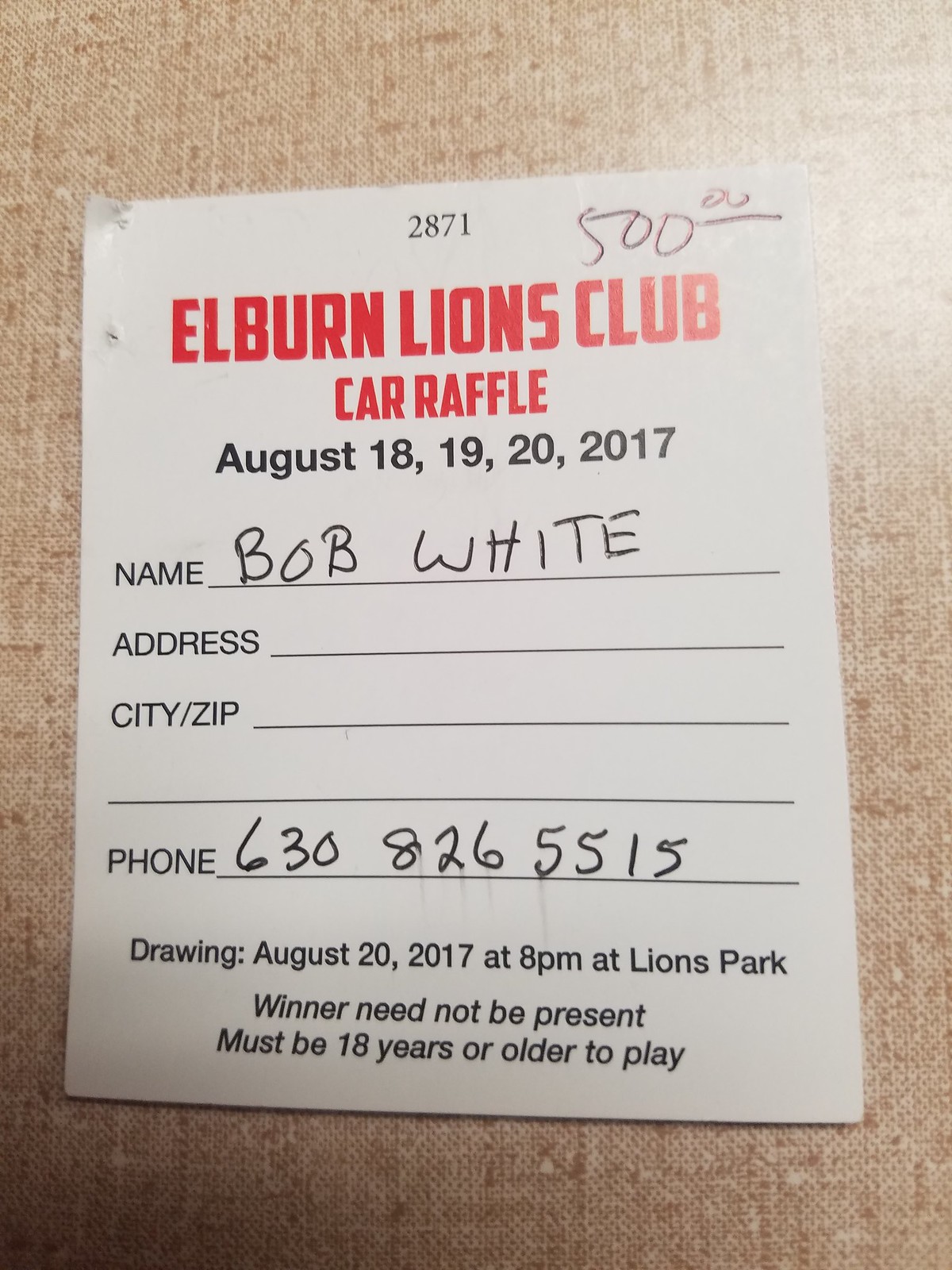In this color photograph, oriented in portrait, a white raffle ticket stub is positioned directly at the center against a beige tweed fabric background. The ticket prominently features the number "2871" at the top, with a handwritten note indicating "$500" in black ink in the upper right corner. Directly below, in bold red lettering, is "Elburn Lions Club," followed by "car raffle" in smaller red text. Further down, in dark black text, the dates "August 18, 19, 20, 2017" are listed. The ticket includes three blank lines for filling out personal information, with "Name," "Address," and "City/Zip." The name "Bob White" is written in black pen on the "Name" line, and a phone number, "630-826-5515," is filled in below. Additional text states that the drawing will be held on "August 20, 2017, at 8 p.m. at Lions Park," specifying that "Winner need not be present" and participants "Must be 18 years or older to play." The image captures the intricate details and layout, emphasizing the structured information and the textured background.